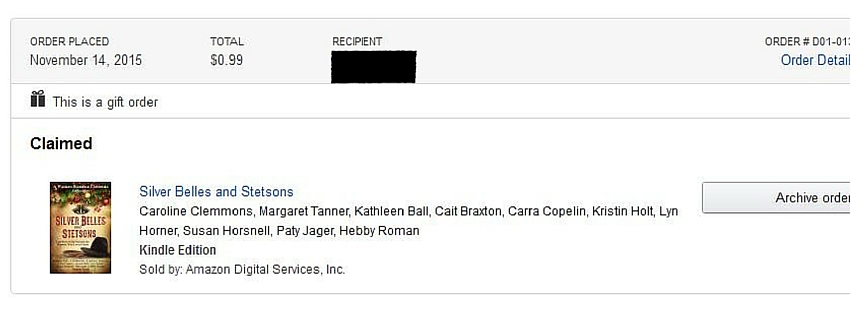A detailed screenshot in landscape mode captures an order confirmation for an Amazon Kindle book. The screenshot is divided into three primary horizontal rows. The top row has a light gray background. In the upper left corner, text reads "Order placed November 14, 2015," while the middle column shows the total amount, "$0.99." The next column displays the word "Recipient," below which is a blacked-out rectangle obscuring the recipient's name. In the upper right corner, the order number "D01/01" is displayed, with an adjacent blue hyperlink labeled "Order details."

The second row begins with a small gift box icon on the left, accompanied by the message "This is a gift order." Beneath this, the word "CLAIMED" is printed in bold black text. 

The third row features an image of a book with a yellow cover. To the right of the image, the book's title, "Silver Bells and Stetsons," is shown in blue text, along with the authors' names: Caroline Clemens, Margaret Tanner, Kathleen Bell, Kate Braxton, Kara Copland, Kristen Holt, Lynn Horner, Susan Horsnell, Patty Jagger, and Hebi Roman. Additional text indicates that this is a Kindle edition sold by Amazon Digital Services. On the far right of the row is a gray button labeled "Archive order."

This screenshot represents an order confirmation for the Kindle book "Silver Bells and Stetsons," placed on November 14, 2015.